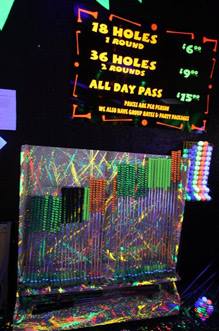The image shows a vibrant, neon-colored sign against a black background, presenting the prices for what appears to be miniature golf. The doorway is adorned with a spectrum of neon lights—yellow, orange, blue, and green—adding to its eye-catching appeal. At the top of the sign, it lists: "18 holes, $6.98," "36 holes, $9.95," and "an all-day pass for $13.94." These prices are low and extraordinary, hinting at a possible retro era, though the usage of neon lights suggests otherwise. The left side of the sign is dominated by yellow text, highlighting the details, while the prices are displayed in green. Additionally, below the pricing, there are mentions of group rates and package deals, though the details are somewhat obscured. Scattered around are neon-colored putters and golf balls, emphasizing the playful, miniature golf theme.